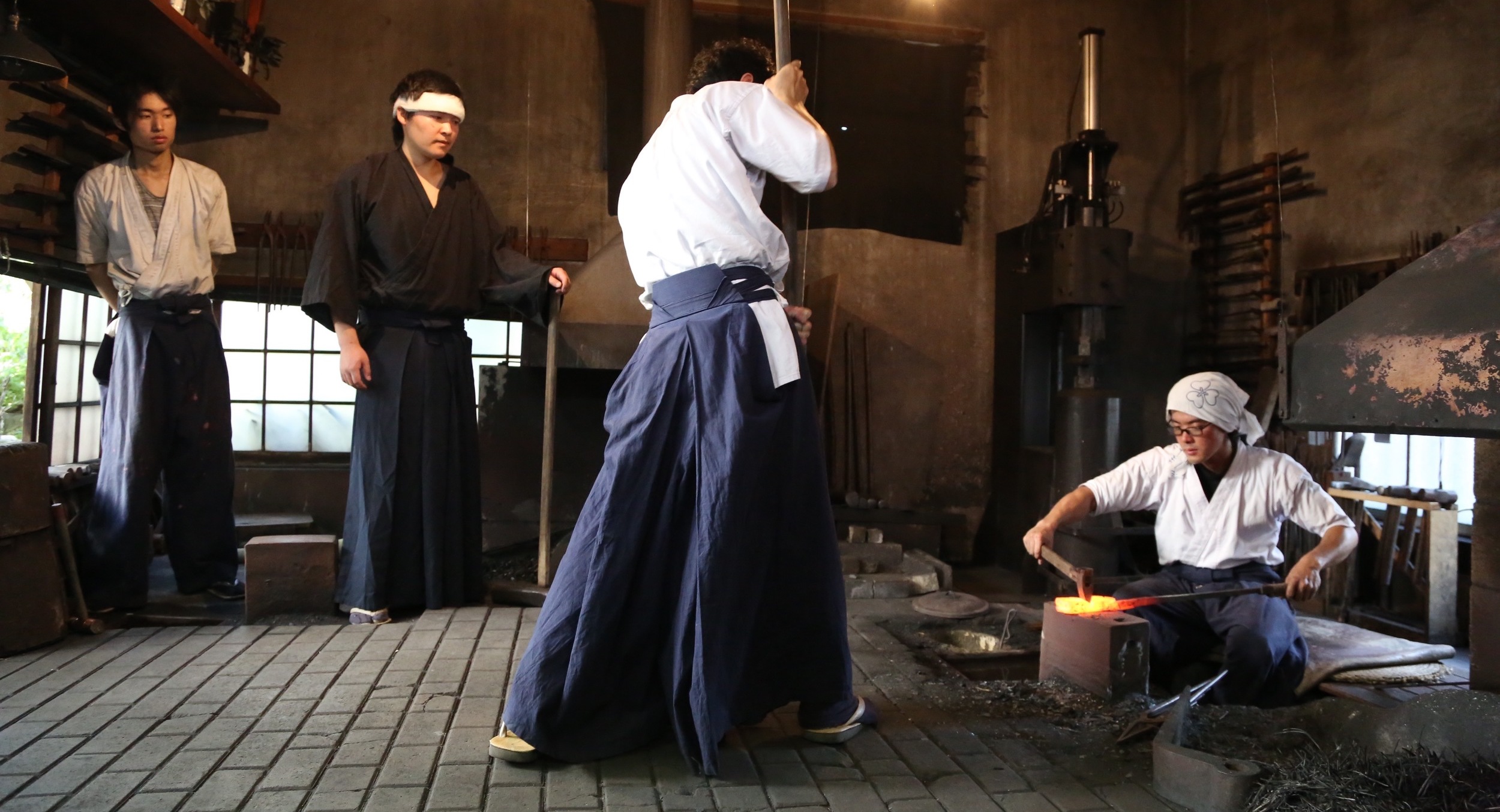In this detailed photograph, four individuals are engaged in traditional Japanese blacksmithing inside a dimly lit smithery. The focus is on the craftsman on the far right, who is seated on the stone floor, intensely working on a glowing orange piece of metal atop an anvil. This individual wears a white bandana with a floral pattern, glasses, a white shirt over a black v-neck, and blue pants. In his left hand, he holds the hot piece of metal while using a hammer with his right to shape it. 

To his left stands another person in traditional Japanese attire - a white shirt paired with blue slacks, holding a tall pole or staff descending from the ceiling. Two additional individuals stand in the background, observing the process. One of these onlookers is dressed in similar traditional Japanese robes with a white top and blue slacks and has short brown hair, while the other is in all black attire with short black hair. The room has several waist-high windows, one of which is open, letting in daylight. The walls are brown, creating a somewhat cramped and dark atmosphere, with various tools scattered around, emphasizing the artisanal activity taking place.